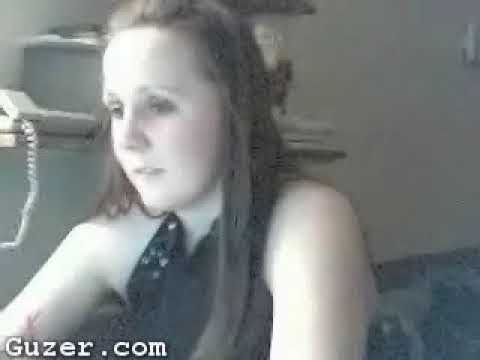The grainy photograph captures an indoor scene featuring a young white woman, possibly in her late teens or early twenties, with long, dirty blonde hair flowing over her black sleeveless top. She has a rosy complexion and fair skin, and she is looking off slightly to the left. Behind her, on her right and our left, there is a built-in wooden shelf attached to a neutral-colored or gray drywall. The shelf holds a white, corded telephone with a springy cord, and other indistinct objects partially obscured by her head. In the lower right corner of the image, there's a hint of a sofa or bedspread with brown and blue tones. Additionally, the bottom left corner of the photo features a small URL in typewriter font that reads "guzer.com."